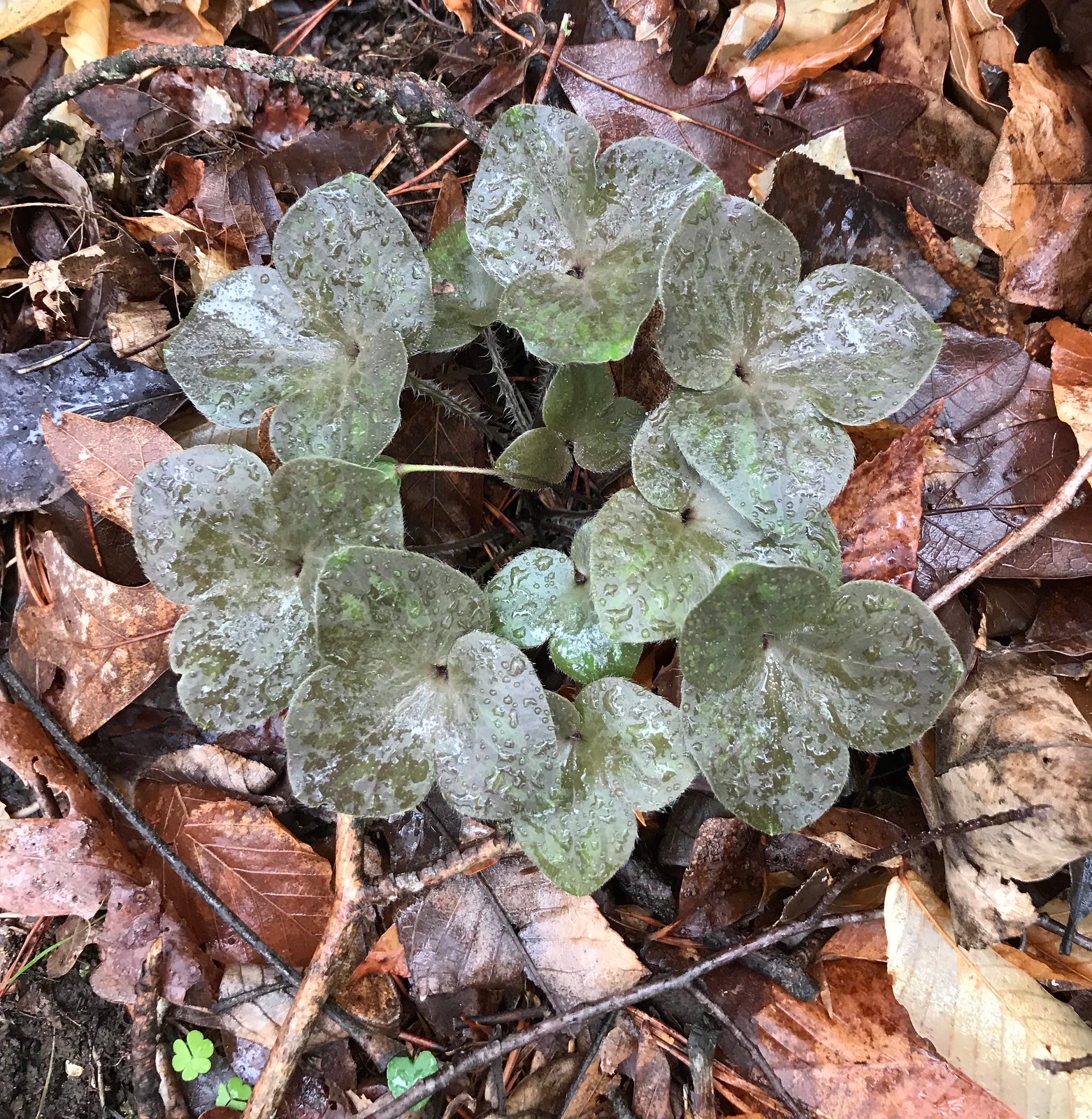The image captures a close-up view of the ground in a natural setting, likely taken during the fall season. Dominating the center of the image is a vibrant green plant with circular formation, characterized by stems each bearing three leaves. Surrounding this central plant are variously colored leaves in shades of yellow, green, orange, and brown, interspersed with twigs and branches, some of which are adorned with moss. The ground around the plant is damp, indicating recent moisture, and small clusters of green clovers are beginning to emerge at the bottom of the scene. This intricate pastiche of autumn elements is artfully arranged, evoking the essence of the season.